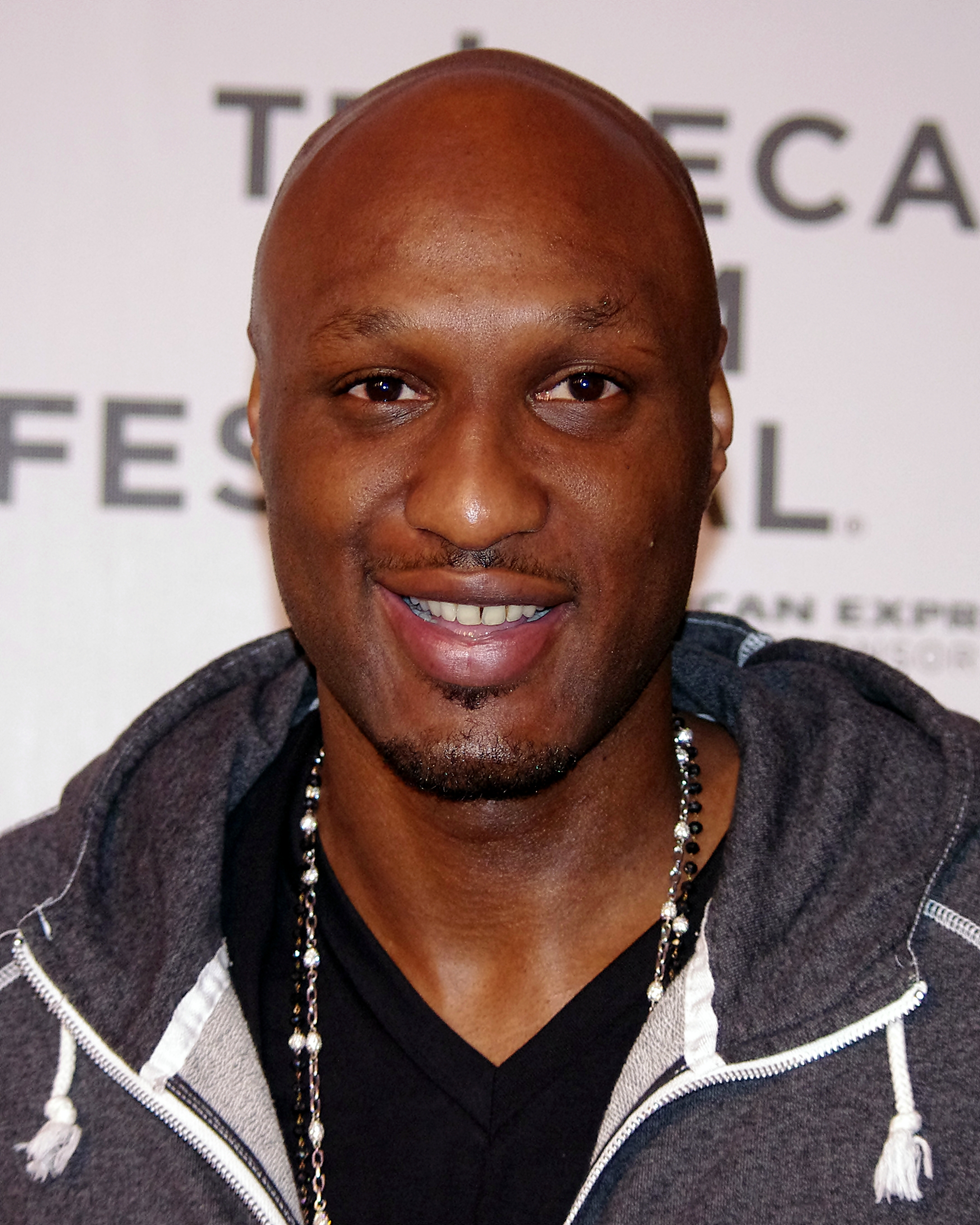This vertically-aligned, close-up photograph captures a smiling man from his chest up, centered in the picture. He has dark skin, a bald head, thin eyebrows, and brown eyes. His smile reveals his teeth, and he has a slight beard and mustache. He is wearing a black v-neck t-shirt under a charcoal-colored, zippered hoodie with white drawstrings. Around his neck are two beaded necklaces, one silver with white beads and the other black with black beads. The background is an off-white or light gray wall with partial text visible, suggesting he is at the Tribeca Film Festival.